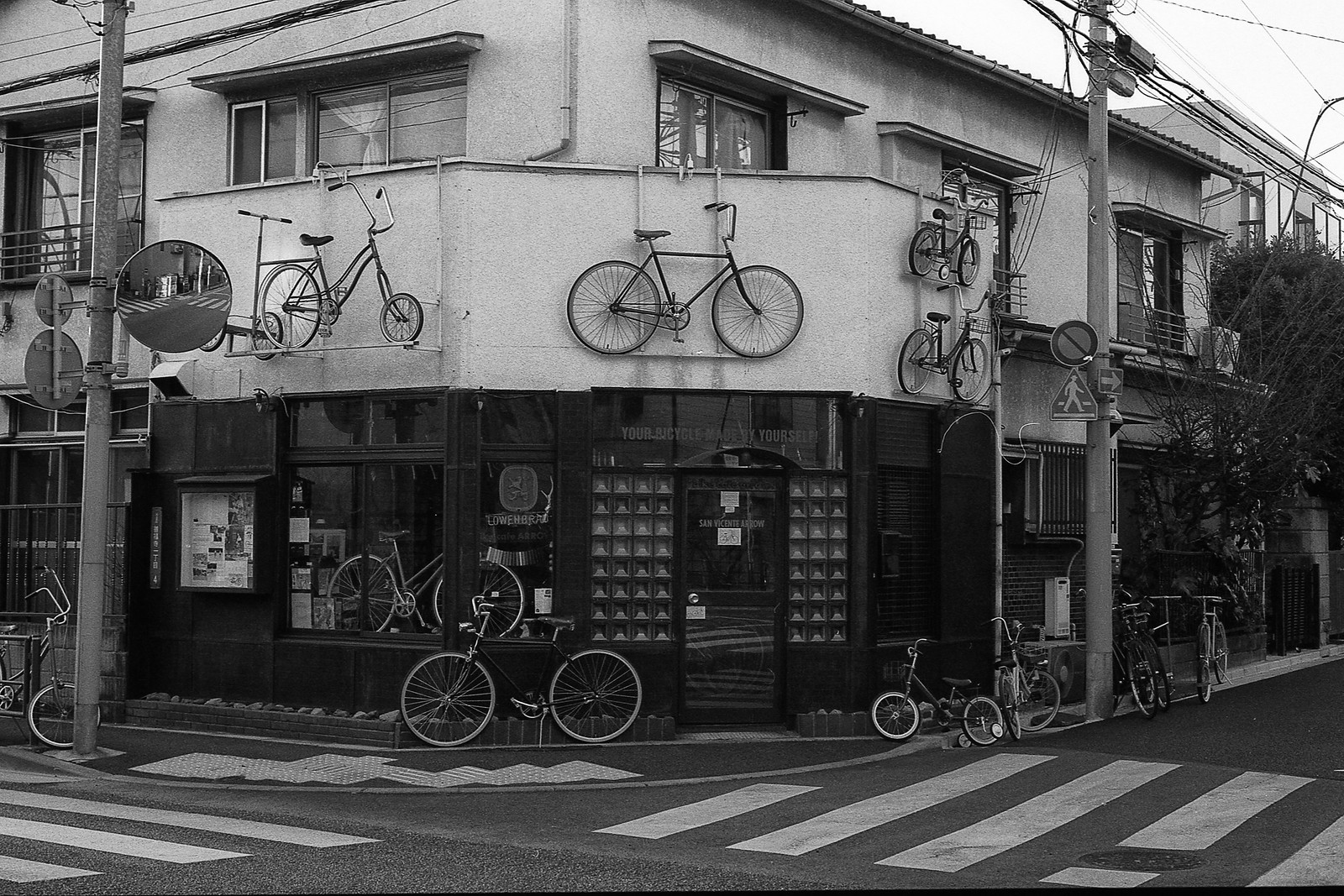This black and white photograph captures a two-story corner storefront, likely a bike shop, situated at the intersection of two streets. The white building front contrasts with the black wooden façade and smoky glass windows. Bicycles dominate the scene, with several mounted on the balcony above the central door—two on each side and one in the middle. Bicycles of various types, including tricycles and those with distinctive banana bars, are parked all around the shop and even visible inside the window. The narrow, rounded sidewalk, due to the building's location on a street turn, has a small pile of snow directly in front of the entrance. 

A pole with a circular traffic mirror and multiple signs, including a pedestrian crossing sign and a no-entry symbol, stands to the left of the building. This side also showcases a notice board filled with various postings. Above the door, windows with awnings suggest that the upper floor may serve as a residential area. Crosswalks marked by white lines are visible on both sides, enhancing the sense of an urban setting bustling with activity.